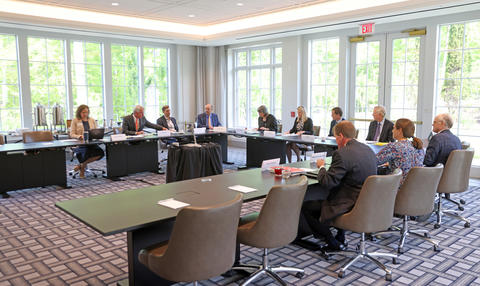The image captures a professional conference taking place in a spacious, well-lit room with floor-to-ceiling windows on both sides, flooding the space with natural light. A u-shaped black table is the focal point, surrounded by brown swivel chairs where around twenty middle-aged professionals, dressed in formal attire such as suits, ties, shirts, and dresses, are seated. Many participants have gray hair, adding to the mature, professional atmosphere. Papers, glasses of water, and some laptops are scattered across the table. The attendees appear engaged in conversation or attentively listening to one another. The room's white walls and ceiling feature a subtle golden or yellow backlighting, complementing the square-patterned blue rug on the floor. Behind one man in the right-hand corner is a red emergency exit sign above a door. Outside the expansive windows, a lush green landscape provides a serene backdrop. This image offers a detailed glimpse into a formal meeting or conference setting in a modern, airy office environment.